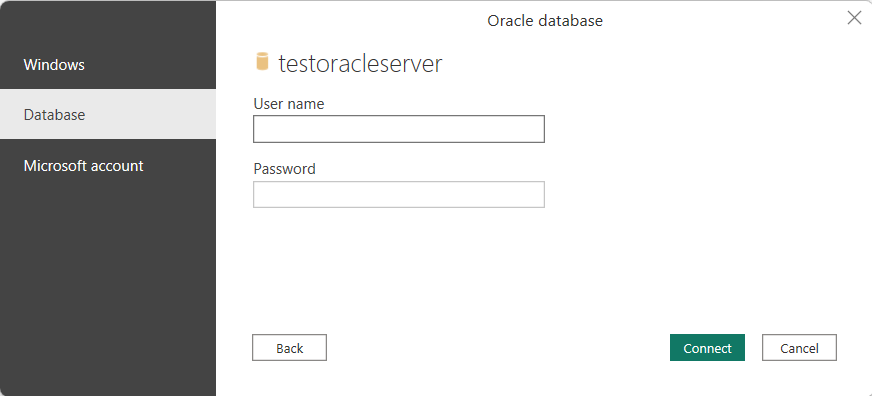The image depicts a login interface labeled as "Test Oracle Server." At the very top of the page, there is a header that reads "Oracle Database." Positioned centrally on the right-hand side is an 'X' button, indicating an option to close the window. On the left side of the page runs a vertical navigation bar with options listed as "Windows," "Databases," and "Microsoft Account."

In the middle section of the interface, prominently displayed, is "Test Oracle Server." Below this title, there are fields provided for the user to enter their username and password. Adjacent to these input fields is a "Back" button, which is styled with a black font and a black outline on a white background.

At the bottom right corner, there are two buttons: a green button labeled "Connect" in white text, and a white "Cancel" button with black font and a black outline. The overall background of the page is white, although the selected "Databases" option in the navigation bar has a light gray highlight.

Next to the "Test Oracle Server" text is a small yellow cylinder icon. The color scheme of the page includes gold, green, black, white, and gray shades, giving a clean and organized appearance. The absence of web address or branding suggests this interface could be a standalone popup, perhaps for user authentication within a larger application.